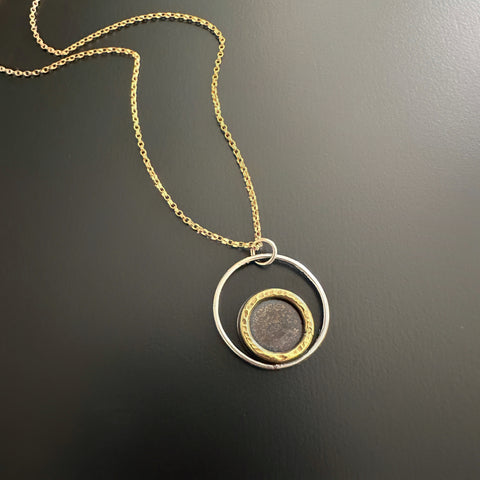This image showcases a gold necklace featuring intricate details against a gradient background that starts light gray at the top and transitions to a darker charcoal color at the bottom. The necklace comprises a fine link gold chain that extends downward from the upper left-hand corner towards the middle of the image. Attached to the chain is a rustic, circular silver pendant. This pendant houses another smaller circular element, consisting of a gold rim encircling a copper piece that resembles an old penny, adding a distinct vintage aesthetic. The interplay of the lustrous gold chain, the aged silver pendant, and the copper centerpiece forms a striking piece of jewelry. The background lacks any text or border, ensuring that the focus remains solely on the necklace with its mix of materials and textures.